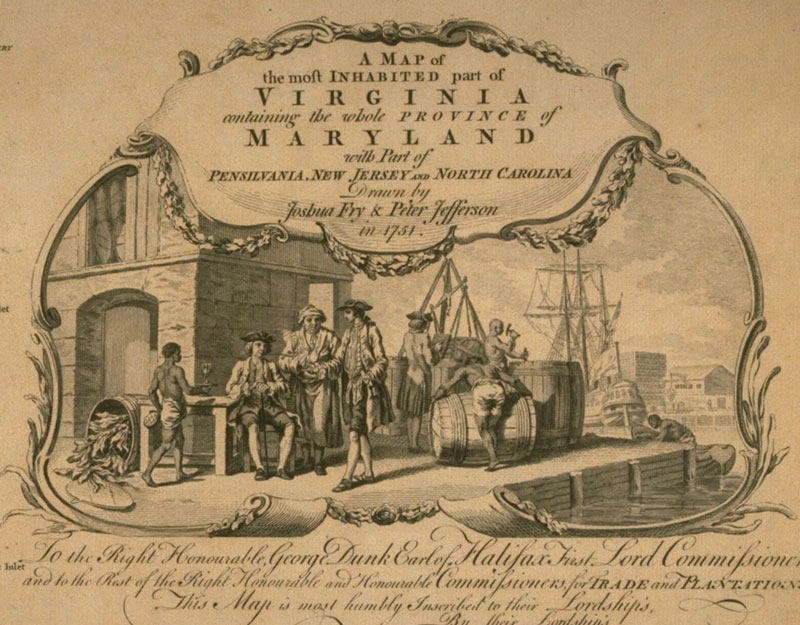This image, reminiscent of an old-fashioned advertisement or news article, appears to be a detailed drawing set atop an aged, yellowing paper. The central scene depicts a bustling colonial seaport dock bustling with activity. On the right, several barrels, including one spilling fish, are scattered along the dock. To the left, a group of men in colonial attire including tri-corner hats and knee-length pants, mill about, some conversing while others work. Among them are black men engaged in labor, moving barrels. In the background, a tall-masted ship looms, though its sails are not raised. Additionally, a house or some structure is partly visible on the left, anchoring the scene in a period setting. The entire image is encased in a Victorian-style frame. Prominently displayed at the top is the text: "A map of the most inhabited part of Virginia, containing the whole province of Maryland with part of Pennsylvania, New Jersey, and North Carolina, drawn by Joshua Fry and Peter Jefferson in 1751," along with smaller, more detailed inscriptions below. The overall impression is one of a historical depiction from the colonial era, capturing the essence and environment of a busy port.